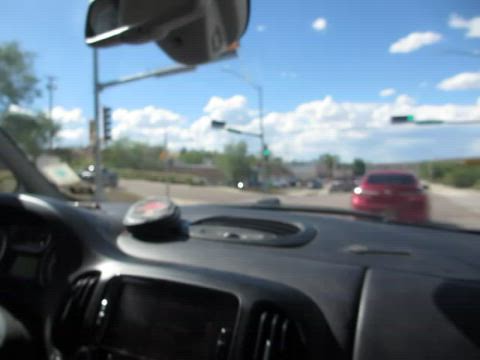A photograph taken from inside a car captures a sunny day through the front windshield. The bottom half of the image is dominated by the car’s black dashboard, featuring a radio media player at the left-center and flanked by air conditioning vents on both sides. A slightly dusty eyeglasses case rests inconspicuously on the dashboard surface. The rearview mirror, situated at the top of the frame, reflects an indistinct image due to the viewing angle. The vantage point from the passenger seat excludes both the steering wheel and the driver from the composition.

The scene outside showcases a clear blue sky adorned with fluffy white clouds, illuminating the surroundings with bright sunlight. Directly ahead, a red sedan waits at an intersection beneath a green traffic light, ready to proceed. Sparse trees are visible in the distance to the left, indicating a possible industrial, business, or retail area. Brick structures or walls are faintly discernible, hinting at nearby buildings. The overall image encapsulates a momentary pause at a traffic intersection, framed by the serene backdrop of a sunny day.